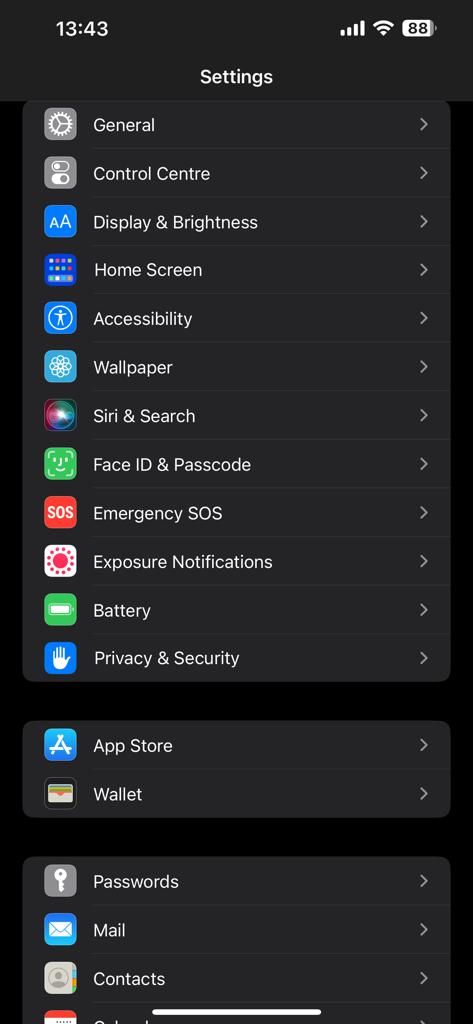The image features a smartphone screen with a predominantly black background. In the upper-left corner, the time is displayed as "13:43" next to icons showing cell signal strength, Wi-Fi connectivity, and a battery level at 88%. Below this, the word "Settings" appears left-justified in white text. 

Adjacent to the word "Settings" is a gear icon. The screen is filled with a list of menu options, each separated by light gray lines and featuring a light gray arrow pointing to the right. Starting from the top, the options listed are: General, Control Center, Display & Brightness, Home Screen, Accessibility, Wallpaper, Siri & Search, Face ID & Passcode, Emergency SOS, Exposure Notifications, Battery, Privacy & Security, App Store, Wallet, Passwords, Mail, Contacts.

The background of the list items is a slightly darker slate gray, which contrasts with the black background behind the entire screen. At the very bottom center of the screen is a white horizontal bar, indicating it can be swiped up to exit the settings menu.

Color accents on the screen include white, black, various shades of gray, with other interface elements highlighted in blue, red, and green.